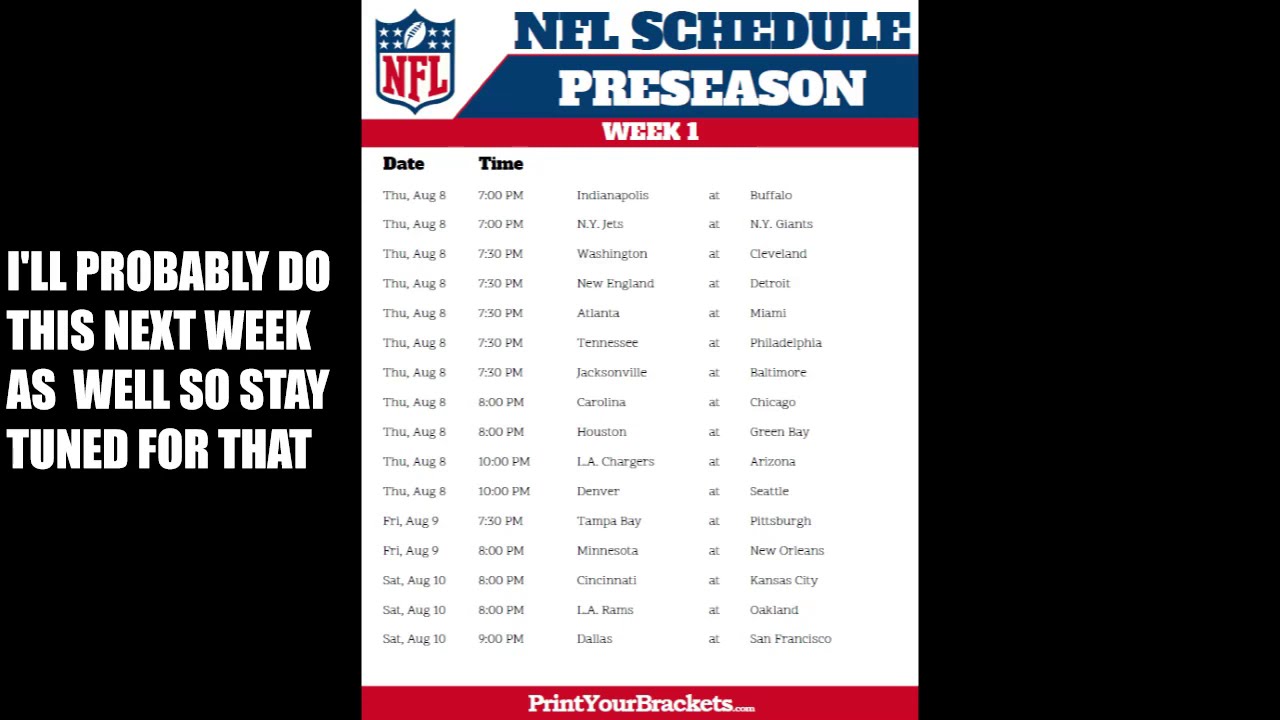The image is a detailed NFL preseason Week 1 schedule chart set against a black background. At the top center, it prominently features the NFL logo and the text "NFL Schedule Preseason Week 1." The schedule is organized into three main columns for the date, time, and the matchup between two teams. The games listed for Thursday, August 8th include Indianapolis at Buffalo at 7 p.m., New York Jets at New York Giants also at 7 p.m., followed by multiple matchups at 7:30 p.m. including Washington at Cleveland, New England at Detroit, Atlanta at Miami, Tennessee at Philadelphia, and Jacksonville at Baltimore. The schedule also includes games for Friday, August 9th, and Saturday, August 10th. The bottom of the chart features white text on a red bar that reads "PrintYourBrackets.com." On the left side, in a black box, it says, "I'll probably do this next week as well, so stay tuned for that." The right side of the image has a black border.